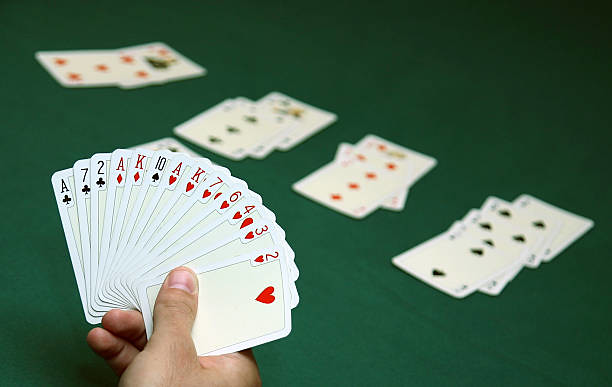A detailed photograph captures a green felt tabletop, typical for card games, adorned with four piles of cards scattered across its surface. In the foreground, a hand elegantly fans out an array of cards, meticulously spaced, suggesting a deliberate arrangement, possibly for a photo shoot or advertisement. The visible cards in the hand include the Ace, Seven, and Two of Clubs; the Ace and King of Diamonds; the Ten of Spades; and the Ace, King, Seven, Six, Four, and Three of Hearts. The background features blurred piles of cards, among which the Three of Clubs and Three of Diamonds are discernible. The overall composition exudes a sense of precision and attention to detail.